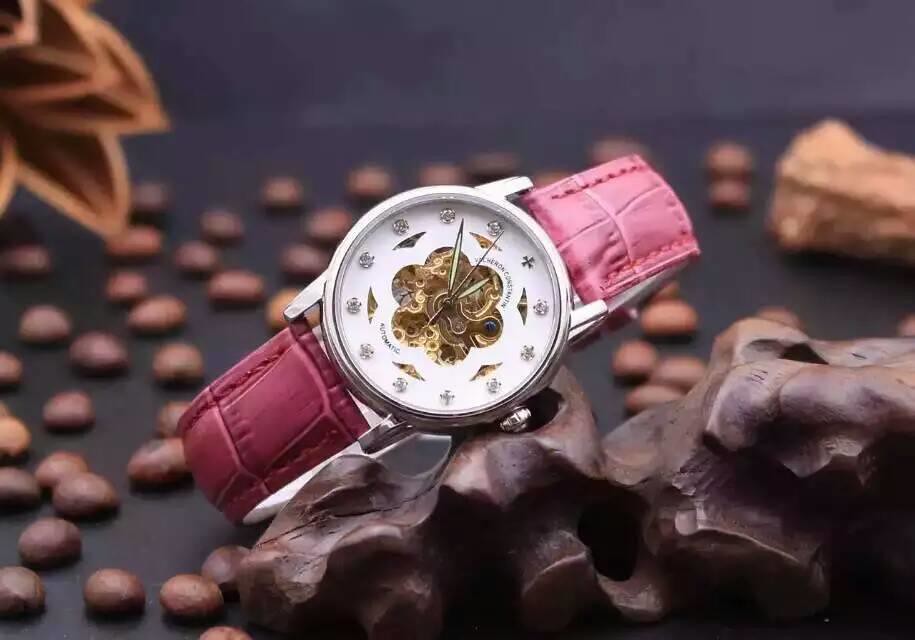This photograph showcases an elegant, close-up view of a luxury woman's watch, presented as part of an advertisement. The watch is meticulously placed atop a mound resembling a sculpture made of rich, chocolate-brown nuts, including visible almond-like nuts and some intricate, flowery elements in the background. 

The watch features a pristine white face with a captivating golden floral-like design at the center, created by intricate golden gears and mechanisms visible through the clear material. The hour markers are adorned with shimmering diamonds, suggesting high-end craftsmanship. The time shown on the watch is precisely 11:52 and 55 seconds. 

Encased in sleek silver chrome metal, the watch exudes sophistication. The hands of the watch are elegantly designed to complement the luxurious look. Adding a pop of color, the wristband is crafted from a reddish leather, almost resembling a hot pink hue. 

Overall, the composition of the photograph underscores the watch's opulent nature, making it a standout piece in any high-end collection.